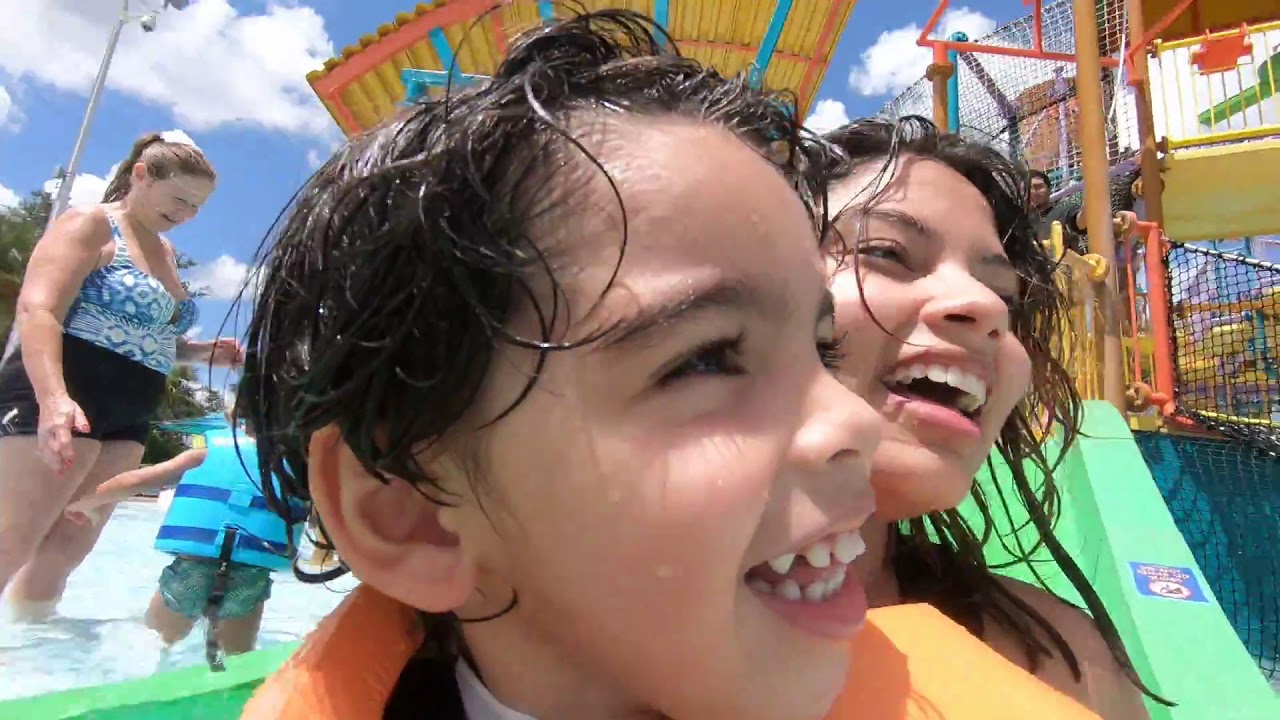The vibrant image captures a joyful scene at a lively water park during the daytime. Central to the image is a young boy, about five or six years old, with black, slicked-back hair and an exuberant, wide smile that reveals his unevenly growing teeth. Clad in a life vest, he is positioned at the forefront, clearly enjoying the thrill of descending a green water slide. Directly behind him is a slightly older female, who could be an older sister or young mother, also smiling with visible teeth, sharing in the fun-filled moment. To the left side of the photo, another touching interaction unfolds: an older woman, possibly in her 50s or early 60s, joyfully looks down at a small child in a light blue life vest, both standing in a small pool area. The background features vibrant water park elements and colorful architecture, punctuated by blue skies with scattered white clouds overhead, enhancing the cheerful and dynamic atmosphere of the scene. An onlooker, possibly a slide attendant, appears behind the prominent pair on the slide, adding depth to this lively snapshot of a fun day out at the water park.